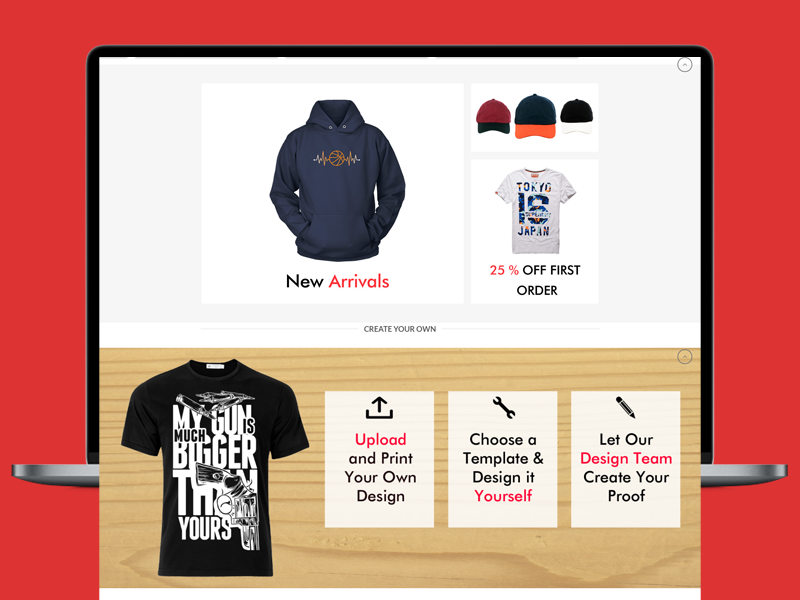This image, likely a screenshot from a website, is rectangular in shape with a red background. At the center, there's an open menu showcasing various design and product options. 

The upper section of this menu features a light gray background displaying a selection of apparel: a dark blue hoodie, three hats (burgundy, dark blue with orange, and black and white), and a light gray t-shirt with blue writing. 

The lower section resembles a blonde wood grain surface and includes more design choices. On the left, there is a black t-shirt with white text referencing guns. To the right, three rectangular options with white backgrounds offer different services: "Upload and Print Your Own Design," "Choose a Template and Design It Yourself," and "Let Our Design Team Create Your Proof."

This detailed composition highlights the variety of customizable apparel and design services available on the website.